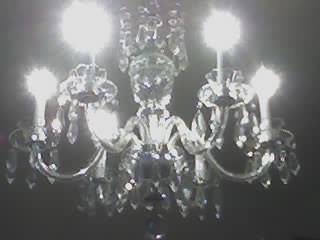This black and white image showcases an elegant chandelier against a dark background. The chandelier features a central crystal base from which five intricately-designed metallic arms extend, curling upwards to support candle-like lights that are lit and appear as large, bright orbs due to the blown-out, overexposed effect of the image. Each arm, adorned with fluted finials, is embellished with shiny, clear crystals hanging delicately from various points, including the center and the arms, adding to its opulent appearance. The tight framing and low resolution of the photograph emphasize the brilliance of the lit chandelier while obscuring the surrounding room, concentrating the viewer's attention on the luxurious details of the light fixture.